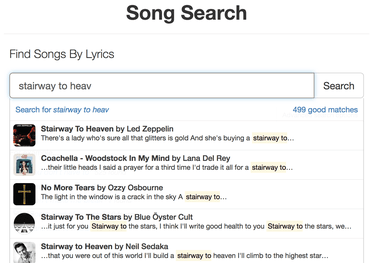**Song Search - Finding Songs by Lyrics**

This screenshot depicts the interface of an app or website named "Song Search," prominently displayed in bold black letters at the top of the page. Underneath the title, a subtitle reads, "Find Songs by Lyrics," followed by a search bar with a "Search" button positioned to its right. The search bar contains the partially typed term "Stairway to Heaven." Immediately below this, a blue hyperlink states "Search for Stairway to Heaven," and to the right of this link, another hyperlink indicates "499 Good Matches."

Below these hyperlinks, a list of song results is displayed. The top entry is "Stairway to Heaven" by Led Zeppelin. The subsequent entries include:
1. "Coachella-Woodstock-In My Mind" by Lana Del Rey
2. "No More Tears" by Ozzy Osbourne
3. "Stairway to the Stars" by Blue Öyster Cult
4. "Stairway to Heaven" by Neil Sedaka

Each song title and artist is clearly listed, providing users with options matching their search query.